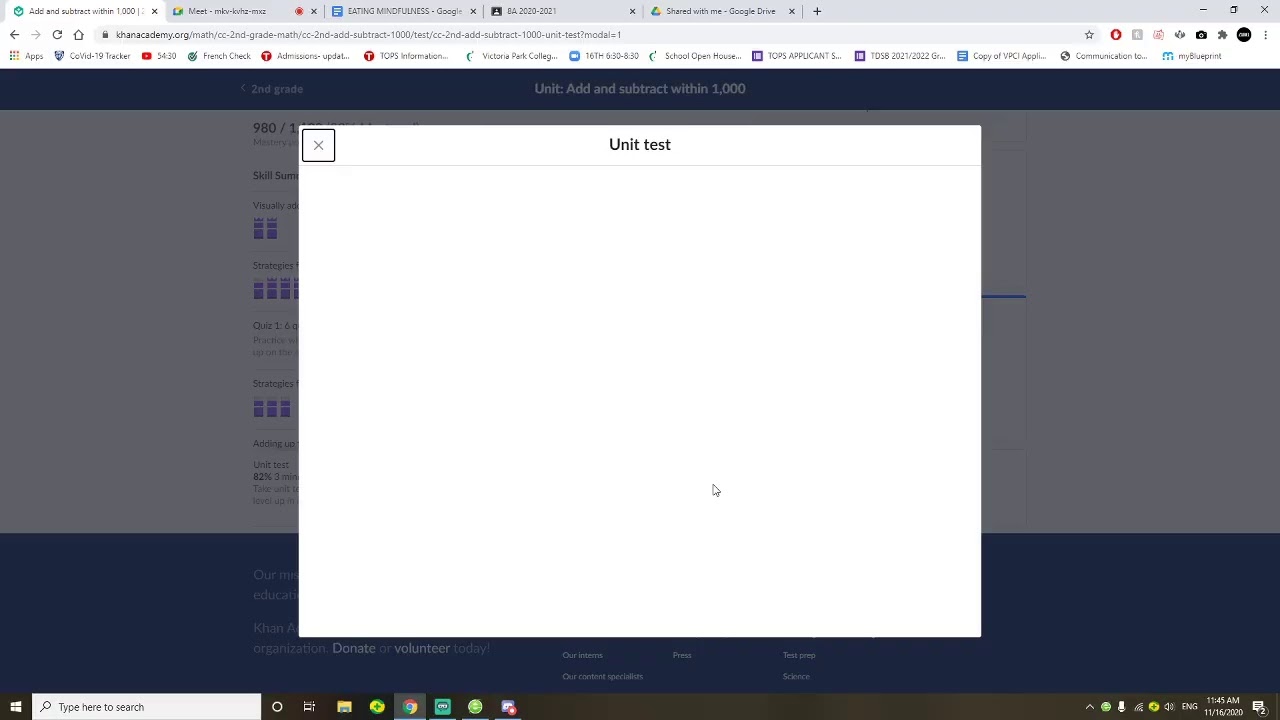This image is a screenshot taken from a computer displaying a browser window with several tabs open at the top, five in total. Among these tabs, one or two are open to Google pages. In the top right corner, you can see the typical browser control buttons: minimize, maximize, and close (X). Just below these, the navigation bar includes a home button and a star icon for favorites. Additionally, there are several other icons, including a red circular button, a camera button, and more.

Below the address bar, a series of saved webpages and apps are visible, including one marked with a shield icon and another with a circle containing the letter "T". Various other items are also saved in this section. A pop-up box appears on the screen labeled "unit test" with a close button (X) on the left side. Behind this pop-up, the text "second grade unit, add and subtract within 1,000" is visible. Additionally, there are some purple bars, likely indicating sections for showing work.

At the bottom of the screen, a search bar that reads "Type here to search" is positioned alongside a Google icon. The current time displayed on the computer is 11:45 a.m.